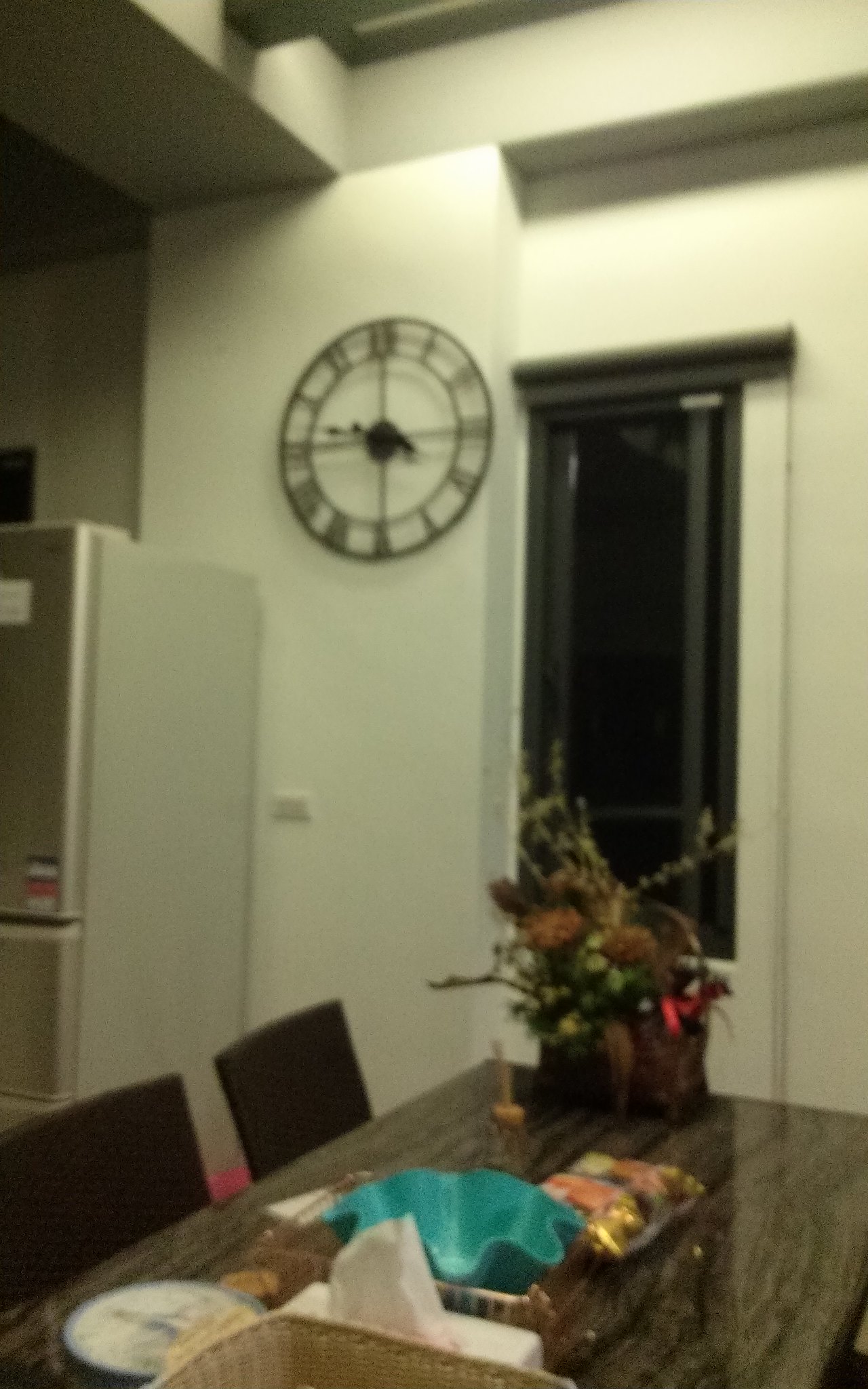In the image, the focal point is a long dining room table, exuding the texture and design of wood. The table is adorned with various decorative and functional items, capturing a homely and inviting atmosphere. Two chairs are neatly pulled up to the table, ready for use. Prominently displayed on the table is a basket filled with vibrant flowers, adding a touch of natural beauty. Towards the center foreground, a seashell-shaped bowl, seemingly part of a snack tray setup, draws attention with its unique design. Nearby, a white dish embellished with a blue pattern and a partially visible woven basket contribute to the eclectic table arrangement. The background reveals a white wall featuring a single window that allows light to filter into the room. Adjacent to the window, a clock is mounted on the wall next to what appears to be a refrigerator, adding functional elements to the cozy dining space.